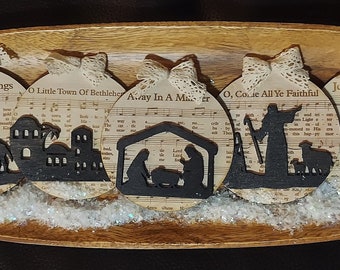The image depicts three circular wooden plaques displayed on a brown wooden shelf, each adorned with Christmas-themed designs and labeled with the titles of traditional Christmas songs. The plaque on the left features the title "O Little Town of Burr Fenton" at the top, a small music note below, and a black silhouette of several houses or buildings and a pine tree at the bottom. The middle plaque is labeled "A Way in a Manger" and showcases black silhouettes of a manger scene, depicting baby Jesus lying in a crib, flanked by Mary and Joseph. The plaque on the right bears the title "O Come All Ye Faithful" and displays a man dressed in a long robe holding a staff, with a large sheep and a baby sheep beside him. Each plaque is topped with a white mesh ribbon or bow tie. The scene has a festive, rustic charm with intricate details highlighting the spirit of Christmas.